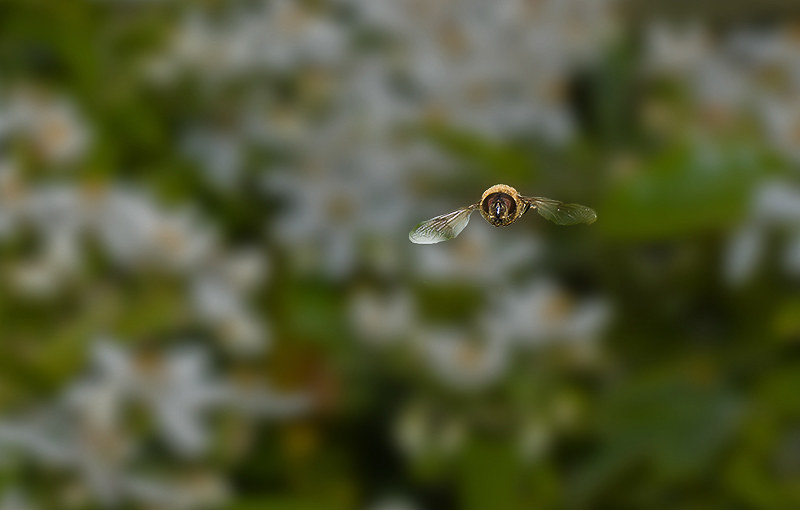The image is a close-up photograph of a bumblebee in mid-flight, taken from the front. The bee is slightly off-center to the right, showcasing its round body adorned with black and yellow markings. Its large eyes are prominently visible, adding to the detail of the shot. The bee's wings are fully spread, with the left wing appearing intact and translucent, while the right wing is slightly damaged with notches. These delicate wings also feature a brownish tint near where they join the body. The background of the image is a blur of green, white, and yellow, suggesting an out-of-focus garden with blooming flowers that have white petals and yellow centers. The overall lighting indicates a bright day, with diffused light likely filtered through clouds or tree leaves, enhancing the vivid details of the bumblebee.